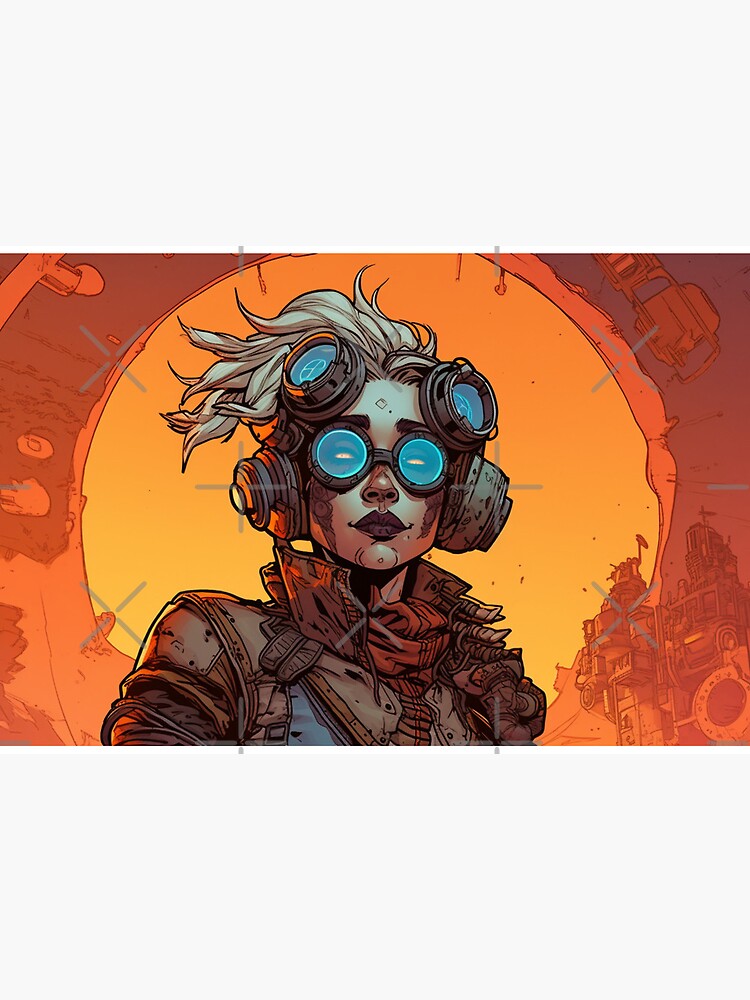The image is an animated drawing of a striking woman with an array of intricate accessories and a distinctive backdrop. She sports a pair of circular, brown-framed goggles with blue lenses, as well as additional singular goggles perched on her forehead and cheek. Her hair, long and white, resembling a windswept mohawk, flows dramatically behind her. Her eyes have a glowing, blue, and sometimes yellowish tint, contributing to her intense gaze. She wears large, thick headphones on the sides of her head, blending seamlessly with her other gear. Her outfit includes a brown leather jacket over a blue shirt, complemented by a red scarf, and she has brown lipstick on. 

In the background, a glowing orange and red industrial scene unfolds, featuring a metallic cityscape and scattered mechanical parts, adding to the dystopian atmosphere. The central figure is framed by an orangey, glowy metal structure and a red-tinted sky or industrial elements, heightening the image's dramatic and futuristic aesthetic. The overall appearance is both captivating and mysterious, with an edgy, post-apocalyptic vibe.